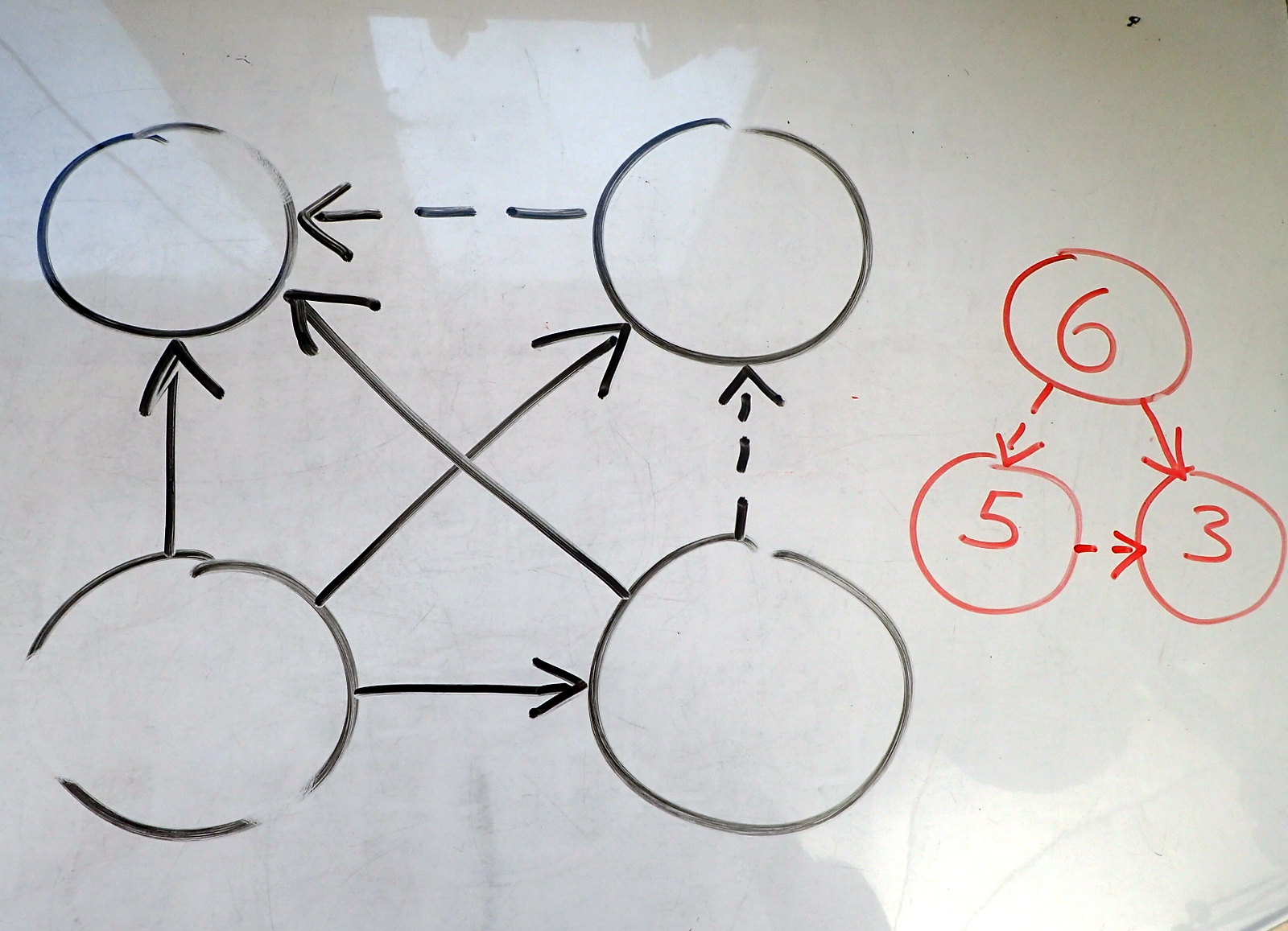The image features a gray piece of paper adorned with intricate drawings in black and red ink. Reflections of two windows and various small objects perched on the window ledges are visible on the paper's surface. Dominating the upper part is a large black circle, positioned directly above another equally large black circle, with a solid arrow linking the bottom circle to the top. To the right of these circles, there is a second pair of large black circles, similarly arranged one above the other. A dotted arrow extends from the bottom circle in this pair toward its top counterpart.

Further detailing these circles, a solid black arrow stretches from the bottom circle of the right pair to the top circle of the left pair, while another black arrow traverses from the bottom circle of the left pair to the top circle of the right pair. Additionally, a dotted arrow connects the top circles of the right and left pairs, and a solid arrow links the bottom circles of both pairs.

Notably, three red circles are incorporated into the diagram: one positioned at the top and two at the bottom. The top red circle is labeled with the number 6 and linked via a dotted arrow to another red circle labeled 5 on the left. This 5-labeled circle then connects via another dotted arrow to a red circle labeled 3 at the bottom right. A solid line also extends directly from the top red circle (6) to the bottom right red circle (3), completing the complex network of connections within the composition.